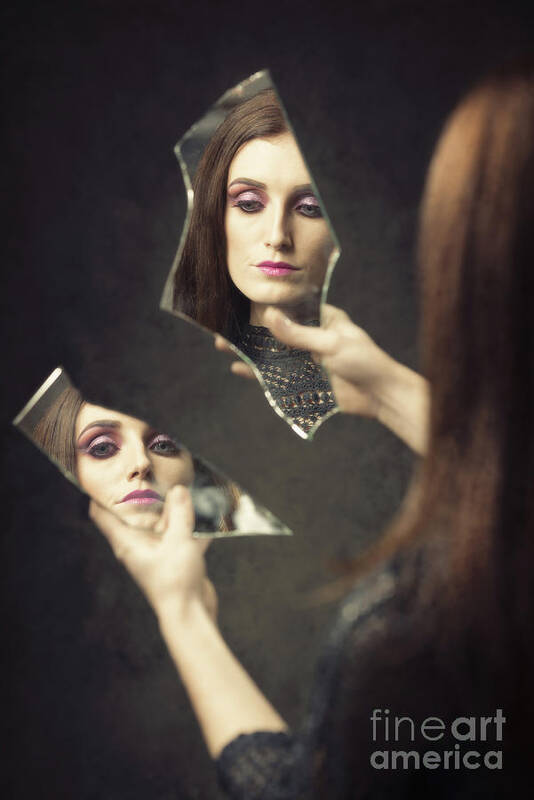The photograph showcases a woman in her mid-20s with long auburn or brown hair, parted in the middle without bangs. Her back is to the viewer as she stands on the right side of the image, facing slightly to the upper left corner. She holds two jagged mirrored shards—one in each hand. The shard in her right hand, raised slightly higher, reflects her calm, downward-gazing face. The shard in her left hand shows a reflection of her face looking directly at the viewer, her eyes conveying a serious and intent expression. She wears heavy makeup, featuring black eyeliner, pink or purple eye shadow, and red or pink lips. Her attire includes a black, lacy-knit top that has a high neckline and extends to the middle of her forearm. The background is dark, fading from black around the edges to brown and gray in the center. The entire image has a photorealistic quality. The "Fine Art America" logo is positioned in the lower right corner.